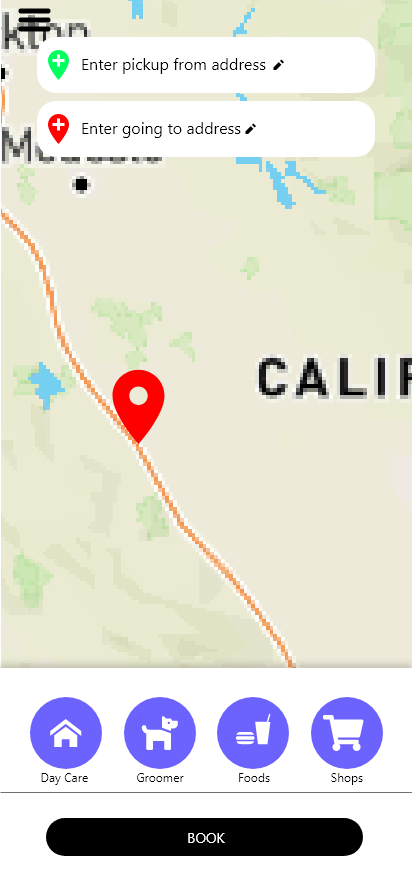This image depicts a screenshot of a mobile app interface, featuring a detailed section of a zoomed-in map. On the right-hand side, the partial text "CALI" followed by the top portion of an "F" suggests the location could be California, though the complete word is not visible due to the cut-off font. In the upper left-hand corner, there are two overlapped white rectangular boxes. The top box displays a green icon resembling a dropper with a plus sign, labeled "Enter pick up from address." Just below, a similar box with a red dropper icon and a white plus sign contains the text "Enter going to address."

At the bottom of the screenshot, a white box houses four purple circles, each representing different service options. The first circle, marked "Daycare," features an icon of a house. The second circle, labeled "Groomer," includes an illustration of a dog. The third circle, tagged "Foods," is accompanied by a burger and a cup with a straw icon. The fourth and final circle reads "Shops," featuring a cart icon. Beneath these service options is a prominent black button labeled "BOOK," indicating the action to confirm or schedule a service.